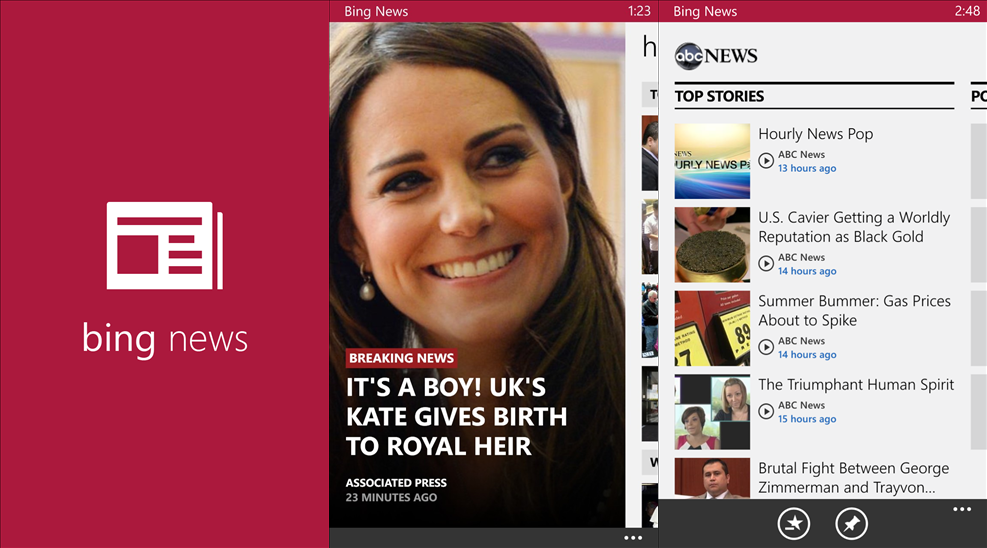In the image, you see a news website, Binknews, displaying several headlines and captions. One of the prominent headlines reads, "It's a Boy: UK Skates Gives Birth to Royal Heir," reported by the Associated Press 23 minutes ago. Other notable headlines on the page include "Top Stories, Hourly News Pop by ABC News," which was posted 13 hours ago. Additional articles featured are "US Caviar Gaining Worldly Reputation as Black Gold," reported by ABC News 14 hours ago, and "Zimmer Bomber: Gas Prices About to Spike," also by ABC News 14 hours ago. Another story titled "The Triumphant Human Spirit" was published by ABC News 15 hours ago, followed by coverage of a "Brutal Fight Between George Zimmerman and Trayvon."

**[Example of a fitting image for the caption:** A screenshot of a news website featuring various urgent and trending headlines, including breaking news about a royal birth, economic updates on US caviar, forecasts on gas prices, and social issues related to a high-profile altercation.]